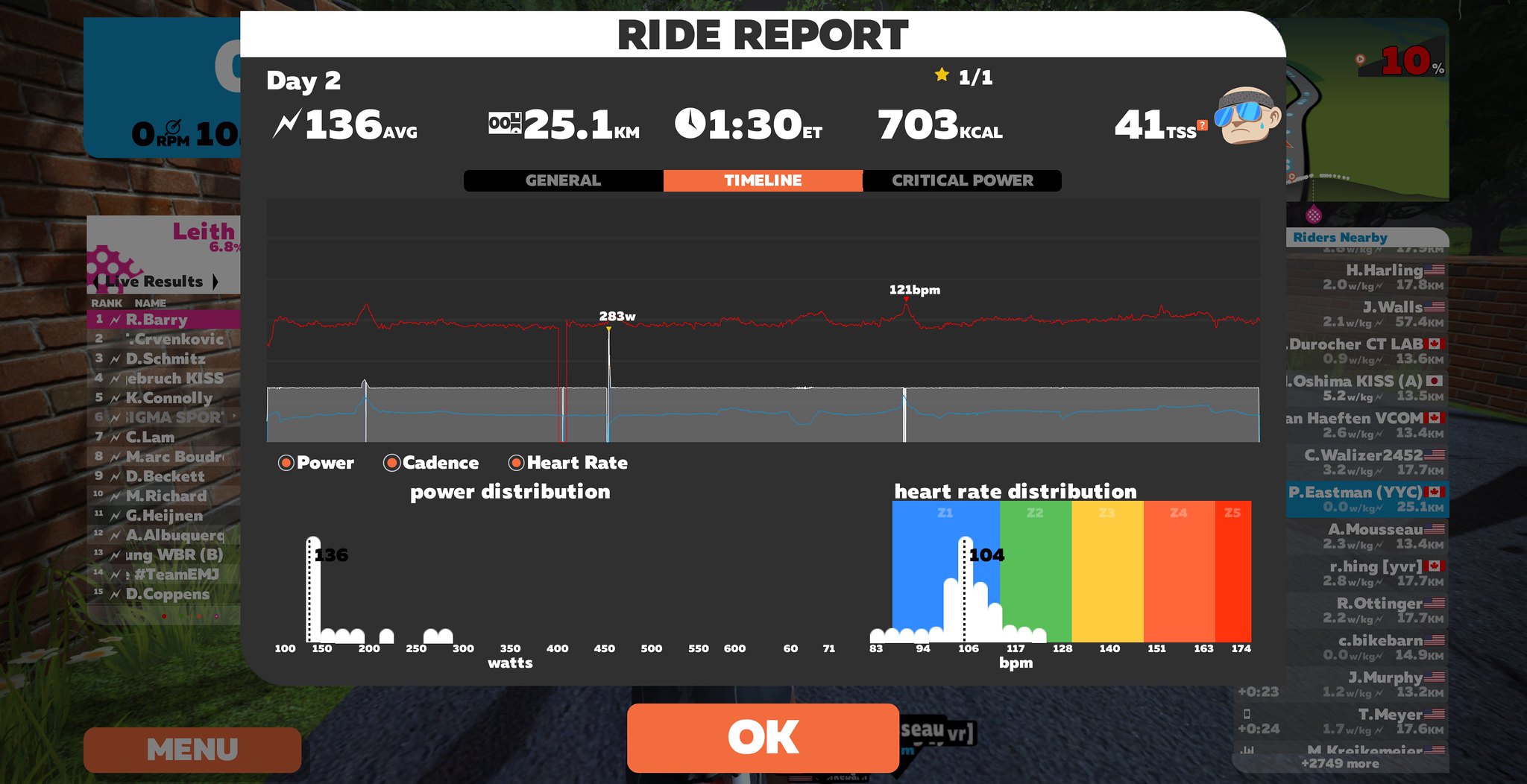This image showcases a digital game interface focusing on a detailed ride report pop-up. The background features a game screen on the left, depicting a brick wall in a grassy area, while the right side lists "Riders Nearby." Centrally, a prominent black wide rectangle houses a white header with the text "Ride Report." Below, details in bold white font read: "Day 2," "1/1," "136 average," "25.1 kilometers," "1:30 ET," "703 calories," "41 TSS," accompanied by an image of a face with sunglasses and a hat. Beneath this, a section titled "Timeline" in orange and white font spans across, with further data showing "Critical Power" and graphical information including a line graph that charts power, cadence, and heart rate over time. Additional metrics include "Power Distribution 136 watts" and "Heart Rate Distribution 104 BPM," with the latter depicted in bar graph form, shaded mostly in blue and green with some yellow and red segments. An "OK" button is located at the bottom right of the report. The background highlights various menus and statistics, though they remain indistinct.